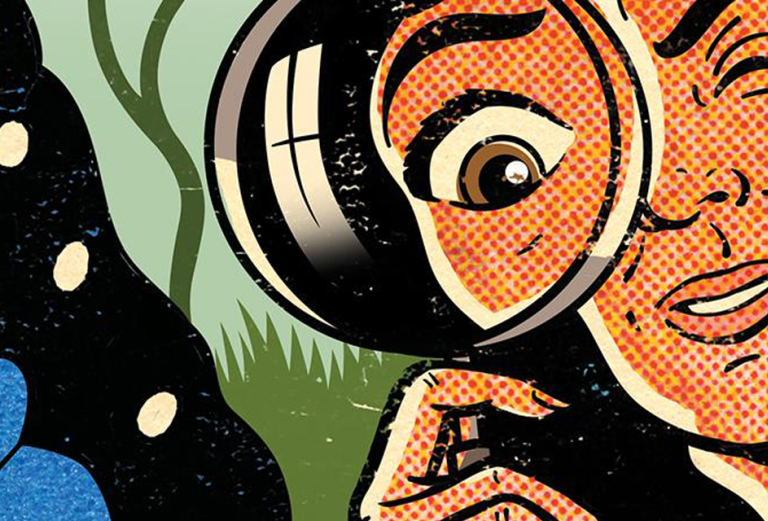The image is a horizontal pop art style illustration featuring a caricature of a person, possibly a lady, holding a magnifying glass over their right eye. Positioned diagonally in the upper right corner, the person's green or yellow face is stylized with a pattern of orange or red speckles, resembling measles. Their right eye, magnified enormously by the glass, shows a detailed brown eye and black pupil, while their left eye is squinted shut. The character has a partial smile and their hand, emerging from the bottom of the image, shows just the index finger extended, with other fingers folded down. The background features graphic elements like green spikes resembling grass, a curvy black space with white dots on the left, and hints of an outdoor scene with a tree and possibly a rock.